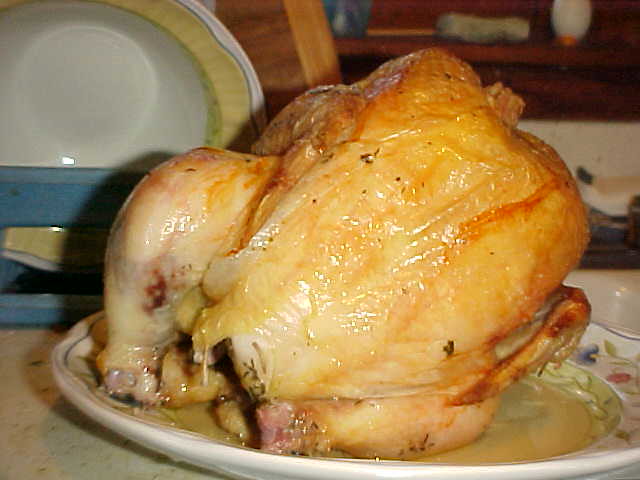The image showcases a large, fully roasted turkey, glistening with a rich orangish-brown glaze. The turkey, succulent and moist, has just come out of the oven and is resting on a floral-designed white plate, immersed in its own savory juices. Positioned prominently in the center, it exudes an appetizing aroma and visually commands the scene. The background features various kitchen elements, including additional plates, possibly on shelves or countertops, and some wood paneling that enhances the warm, homely atmosphere. The image appears to have been taken with a flash, as the details of the turkey and the background objects are sharply illuminated. The white countertop beneath the plate further accentuates the vibrant colors of the roasted turkey, making it even more inviting.